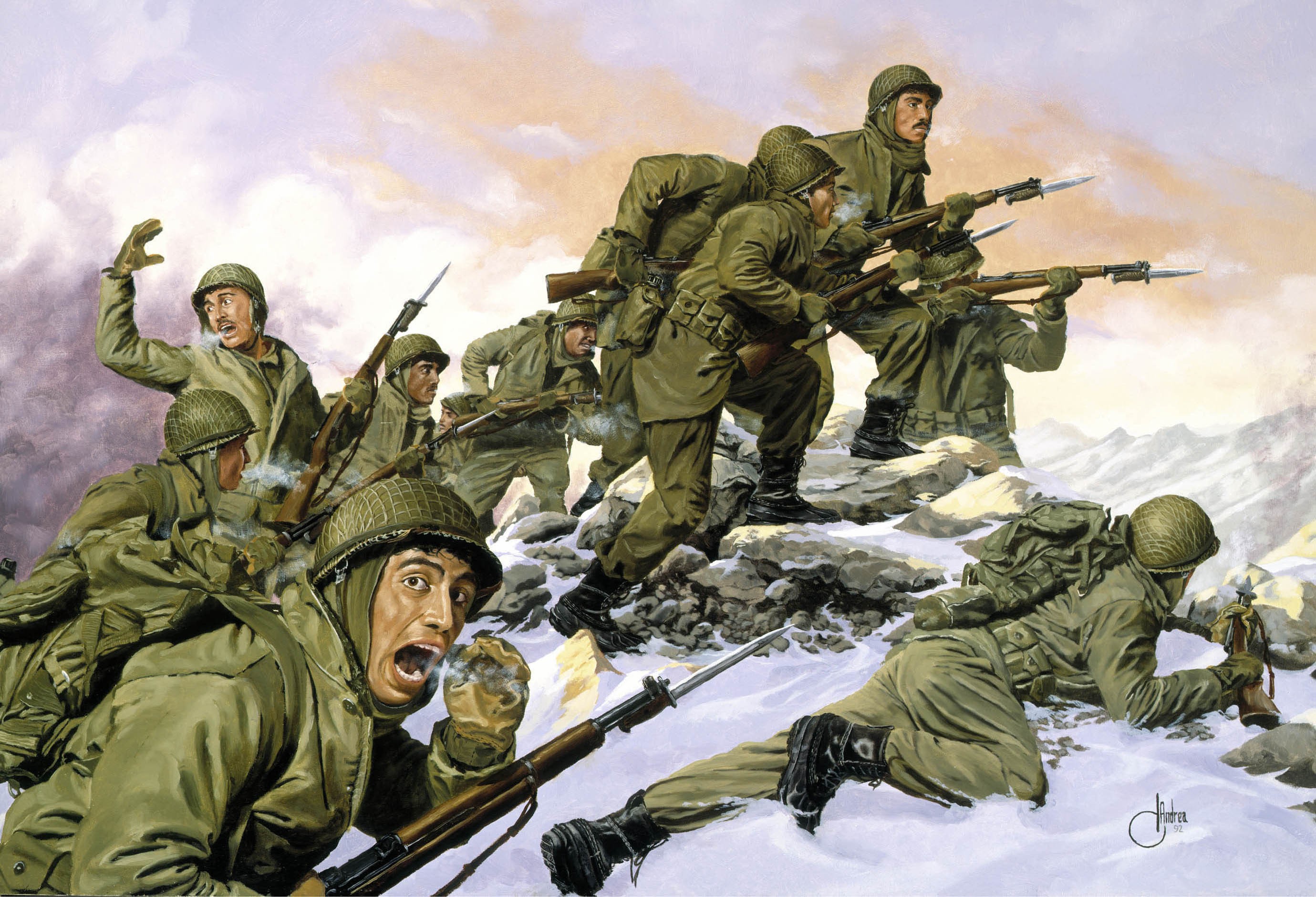The artwork is a detailed winter scene depicting about 10 soldiers in green military uniforms, moving over the snowy, rocky crest of a hill. These soldiers, possibly South Asian, are equipped with army green bowl helmets and black strapped faces, and they all wear black boots. Each soldier holds a bolt-action rifle, complete with a metallic bayonet affixed to the wooden brown stock of the gun. One soldier stands out, smoking a cigar with white smoke visible around his open mouth, emphasizing the cold atmosphere. Another soldier is depicted in a prone position on the hillside, seemingly assessing the enemy below. Their visible breath further accentuates the frigid temperatures. In the background, towering snow-capped mountains line the horizon under a cloudy sky tinged with hues of white, gray, light brown, and orange. The detailed rendering suggests a dramatic charge forward or preparation for a defensive stance, captured beautifully, likely through an oil painting technique.